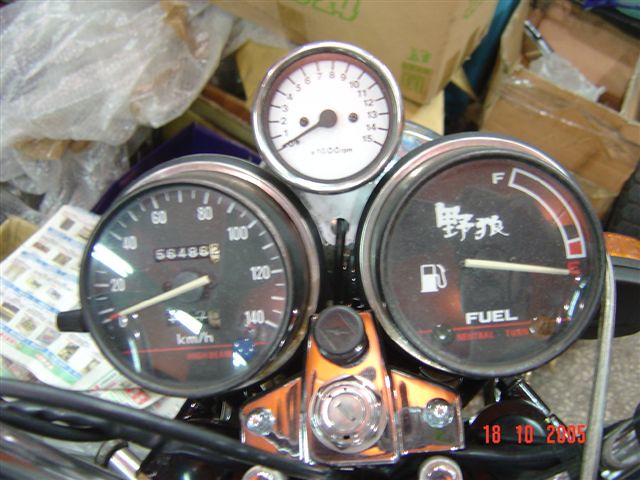This photograph, likely taken with a Polaroid camera as suggested by the bright red date "18-10-2005" imprinted on it, captures a detailed view of a set of motorcycle gauges inside a cluttered garage. The overall quality of the image is slightly blurry, consistent with many older photographs, enhancing its vintage feel.

The background features cardboard boxes scattered around and several magazines or catalogs piled in the back left corner, emphasizing the typical disorderly environment of a working garage. 

The focus of the image is on three primary gauges mounted on the motorcycle. The two larger gauges, with black backgrounds, flank a smaller, centrally positioned white gauge. The left larger gauge, calibrated in kilometers per hour, displays an odometer reading of 66,486.2 km along with an unspecified indicator obscured by glare. The right larger gauge is a fuel meter, notable for containing Kanji characters, thereby suggesting that the motorcycle is of Japanese origin. This gauge currently indicates that the fuel tank is empty. Positioned above and between these two gauges, the smaller top gauge reads RPM, ranging from 1 to 15.

The motorcycle's head, where the handlebars converge, is coated in a unique bronze-orange hue, contrasting with the black handlebars visible at the very bottom of the image. The photograph is taken from a slightly top-down perspective, capturing the gauges prominently along with a hint of the handlebars and head of the motorcycle.